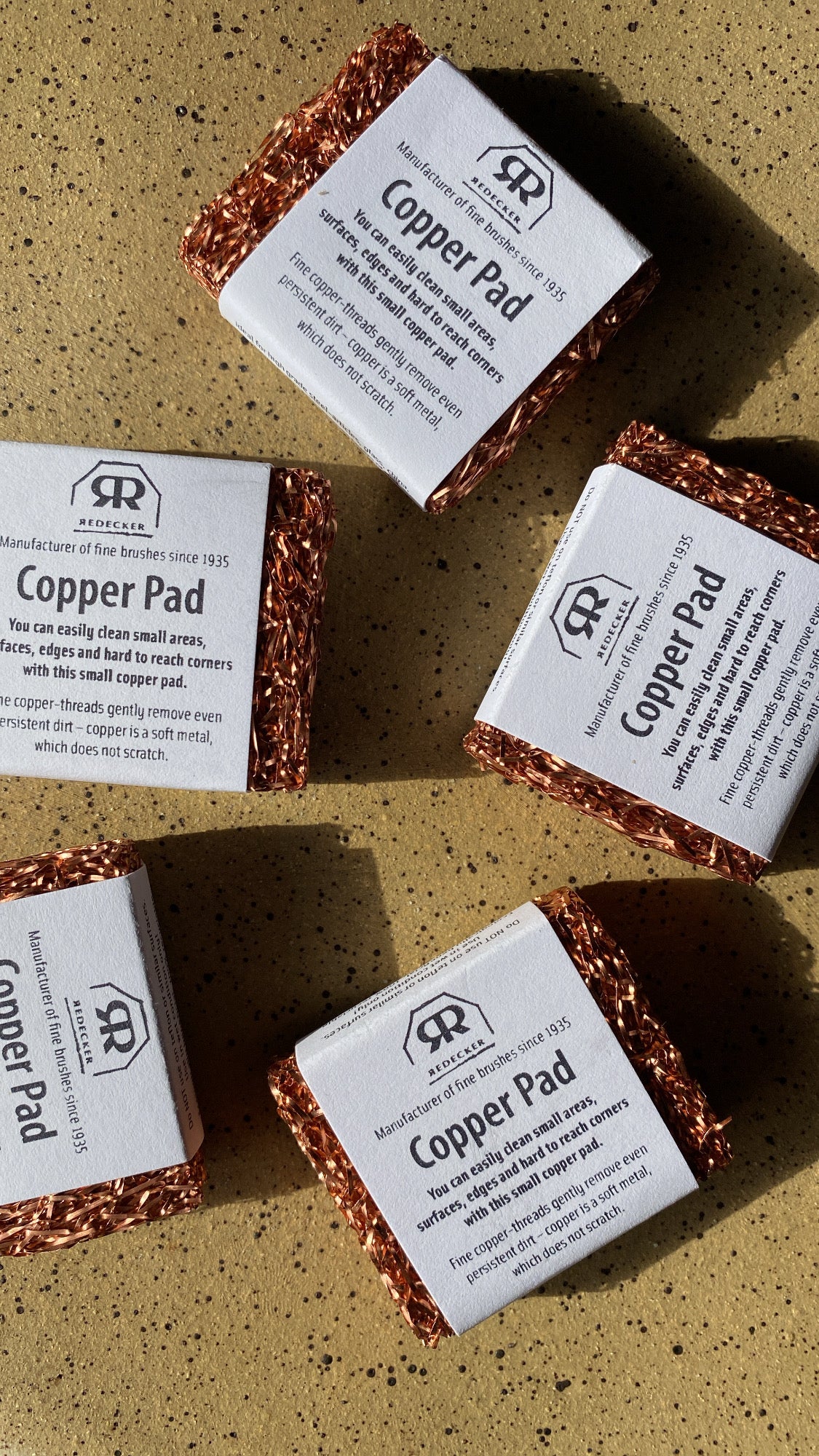The photograph showcases five copper scouring pads arranged on a yellow countertop with small black specks. Each square-shaped pad is packaged in a white paper band that prominently displays the brand "REDECKER" along with the text "Manufacturer of fine brushes since 1935." These labels, which wrap around the pads, indicate the product name "Copper Pad" and provide a detailed description: "You can easily clean small areas, surfaces, edges, and hard-to-reach corners with the small copper pad. Fine copper threads gently remove even persistent dirt. Copper is a soft metal which does not scratch." The pads are positioned with two stacked in the center, two angled on the right, and one on the left, casting slight shadows on the countertop.